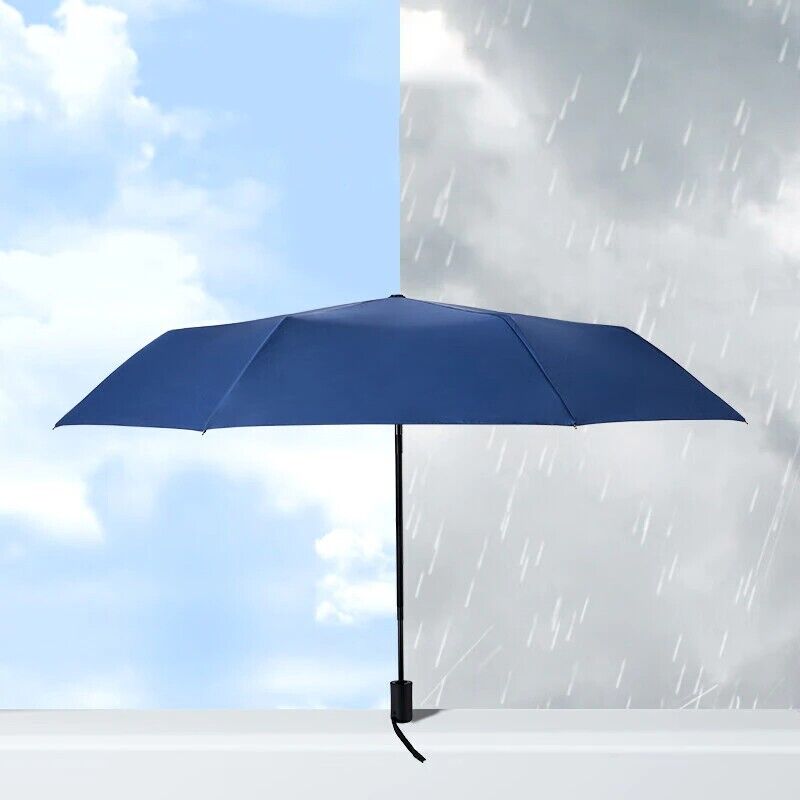The image is a digitally generated art piece with a strong visual contrast. At the bottom, there is a light gray, almost white, banister or window pane. Perfectly balanced at the center of this platform, there stands an open umbrella with a thin black handle and pole, featuring a navy blue canopy. The striking element of the piece lies in its background, which is split down the middle. 

The left half depicts a clear, sunny day with a light blue sky and fluffy white clouds, suggesting a perfect, sunny weather. In contrast, the right half shows a medium gray sky with light gray clouds and white raindrops falling, creating a stark juxtaposition. The duality of the weather in the background encapsulates the theme of contrasting atmospheres, making it a fascinating and visually compelling piece.